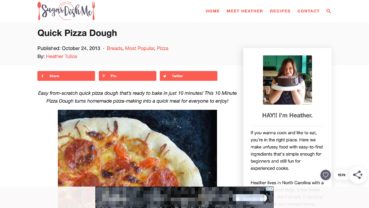In this image, we observe a screenshot of a recipe page from a website. The logo in the upper left-hand corner appears to spell out "Sugars Dosh Me," although it is somewhat blurry and difficult to read clearly. In the upper right portion of the website, there are various buttons.

The title of the recipe prominently displayed at the top reads "Quick Pizza Dough," and it was published on October 24th, 2013. The author's name, Heather, is listed just below the title. There are three buttons situated before the recipe content begins. A small line of text under the title describes the recipe: "A 10-minute pizza dough turns homemade pizza making into a quick meal for everyone to enjoy."

An image of the pizza is also featured within the post.

On the right side of the webpage, there is a dedicated section for the author. It includes a photo of Heather and an introductory line that reads, "Hey, I'm Heather." Beneath her picture, there are a couple of paragraphs presumably written by Heather, offering more about herself or the recipe.

The overall layout provides a user-friendly interface, combining visual and textual elements to guide the reader through the recipe efficiently.